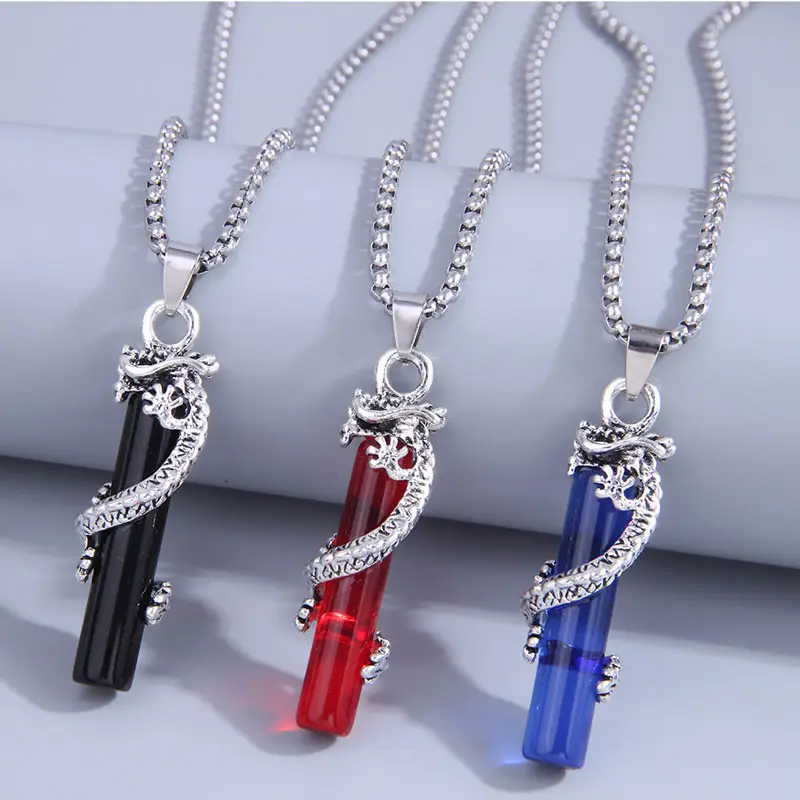In this image, a pristine white, cushiony support tube displays three pendants in a visually appealing arrangement. Each pendant is crafted with a silver dragon coiled meticulously around a glass vial, giving the impression of protecting the precious contents within. The pendants are draped elegantly over the support, held securely by a thick, silver chain. The display emphasizes the unique color of the liquids within each vial: the first houses an opaque black liquid, the second a vivid red, and the third a striking blue. The dragon's head on each pendant forms a silver clasp that connects to the chain, providing both functionality and intricate detail. This setup creates an enchanting product presentation, evoking the mystique of potent, magical potions.